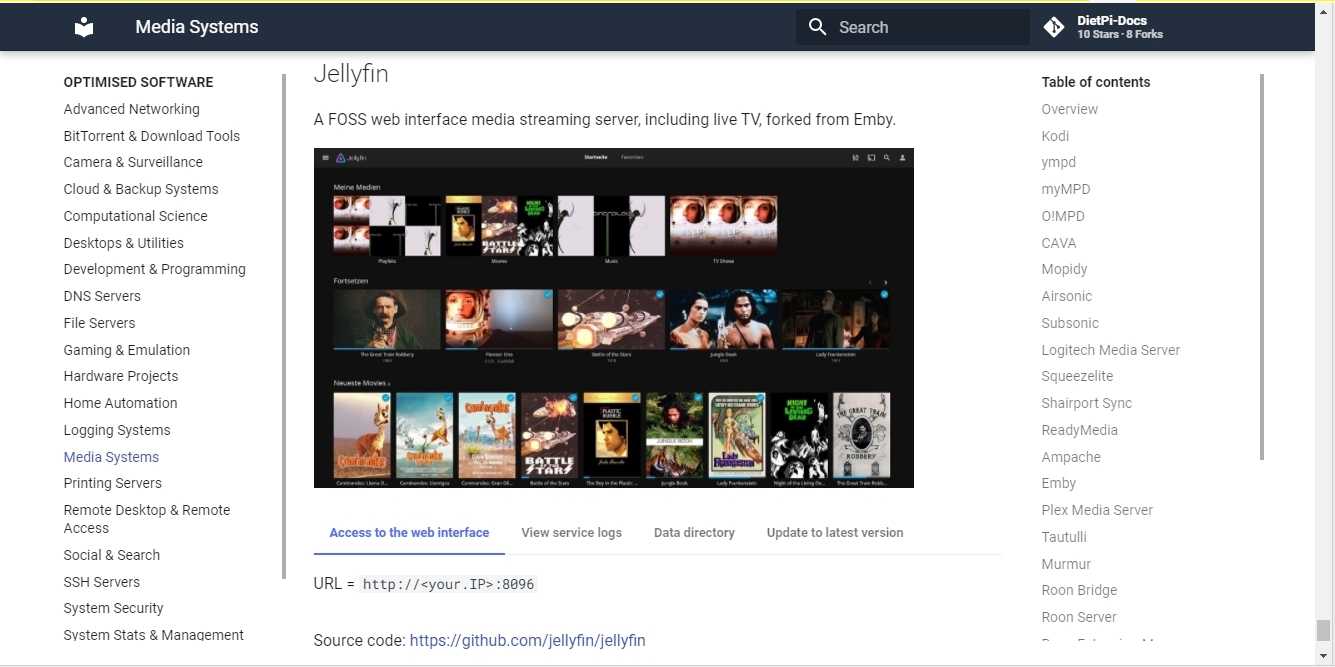This detailed and thorough descriptive caption captures all the elements present in the given screenshot:

---

The screenshot features a user interface with a black horizontal header at the top.

- On the left side of the header, there is a white square with a white circle positioned above it.
- To the right of this icon, the text "Media Systems" is displayed.
- Slightly right of the center, there is a white magnifying glass icon. The word "Search" is written in gray text to the right of the magnifying glass.
- On the far right side of the header, there is a white triangle containing black lines inside it. To the right of this triangle, the bold white text reads "Docs," beginning with the letter 'D'.

Below this header, on the left side, bold black text reads "Optimized Software," followed by a long list extending down to the bottom of the screen.

To the right of this list, there is a vertical gray line separating it from the other content.

On the far right side, in the top section, gray text reads "Jellyfin."
- Two lines below this, a description reads "A FOSS WEB INTERFACE MEDIA STREAMING SERVER INCLUDING LIVE TV FORKED FROM MB."

Below this description, a black rectangle contains several squares with various images inside.

Further to the right, in the top right corner of the screen, bold black text reads "Table of Contents," and below this title is a list in gray text.

---

This caption provides a detailed and precise description of each element visible in the screenshot.